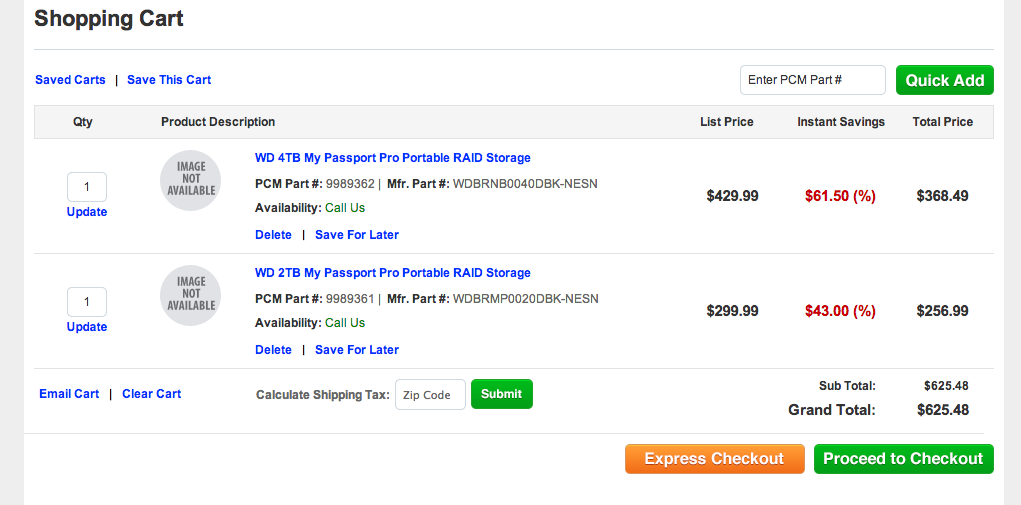This screenshot captures an online shopping scenario with a detailed user interface layout. The left and right sides of the screenshot have a light gray border approximately half an inch wide, while the rest of the background is white.

In the top left corner, just inside the gray border and within the white area, the bolded text "Shopping Cart" is prominently displayed. Below this header, a thin blue line extends horizontally across the screen. 

Underneath this line, on the left side, bold blue text reads "Saved Carts." This section is separated from the next by a black line, beneath which "Save This Cart" is written. On the right side, a green tab with bolded white text says "Quick Add," flanked by a white tab with a small black border that reads "Enter PCM Part Number" in black text.

Further down, a light gray bar about half an inch thick runs horizontally. It features the column headers: "Qty" (Quantity) on the left, "Product Description" next to it, and from right to left: "Total Price", "Instant Savings", and "List Price".

The main section lists two items. Each item entry consists of:
- A small square with a number representing the quantity, accompanied by an "Update" link in blue below it.
- A placeholder profile image that is gray with the text "Image Not Available".
- The product name in blue, followed by the PCM part number.
- A separator line, underneath which the MFR part number is given, with a note stating "For availability, call us" for both items.
- Below this, blue "Delete" and "Save for Later" options are provided for each product.

Under the "List Price" section, the prices are listed with "Instant Savings" shown in red, indicating the amount saved. The "Total Price" column reflects the final price.

At the bottom left of the screen, there is a blue "Email Cart" link followed by a black line with the "Clear Cart" option below. Additionally, there is a section for calculating shipping tax where users can enter their zip code. This section has a green tab with white lettering for submission.

On the right side:
- The "Total," "Subtotal," and "Grand Total" are calculated and displayed.
- In the bottom right corner, a long green rectangular tab with "Proceed to Checkout" is shown, and to its left, an orange tab reading "Express Checkout". 

This comprehensive layout provides a detailed overview for users managing their online shopping carts.